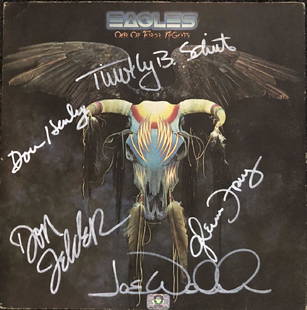This is an image of a signed album cover by the band Eagles. The background is very dark, almost black, giving it a somber, mysterious atmosphere. At the top of the image, "Eagles" is prominently displayed in slightly blurred silver lettering, adding a special effect that draws the eye. The central figure on the album cover is a surreal composite: it features an angelic form with wings juxtaposed with bull horns, possibly resembling a cow skull, adding an intricate, almost trick-effect design element. Dangling feathers or hair from the figure add to the ethereal and complex visual. Autographs from the band members are scattered across the cover in white ink. Notable signatures include Glenn Frey on the right side, Joe Walsh at the bottom, and another member with initials TBS at the top. Overall, the image conveys a vintage, iconic feel with layered elements and distinctive signatures.